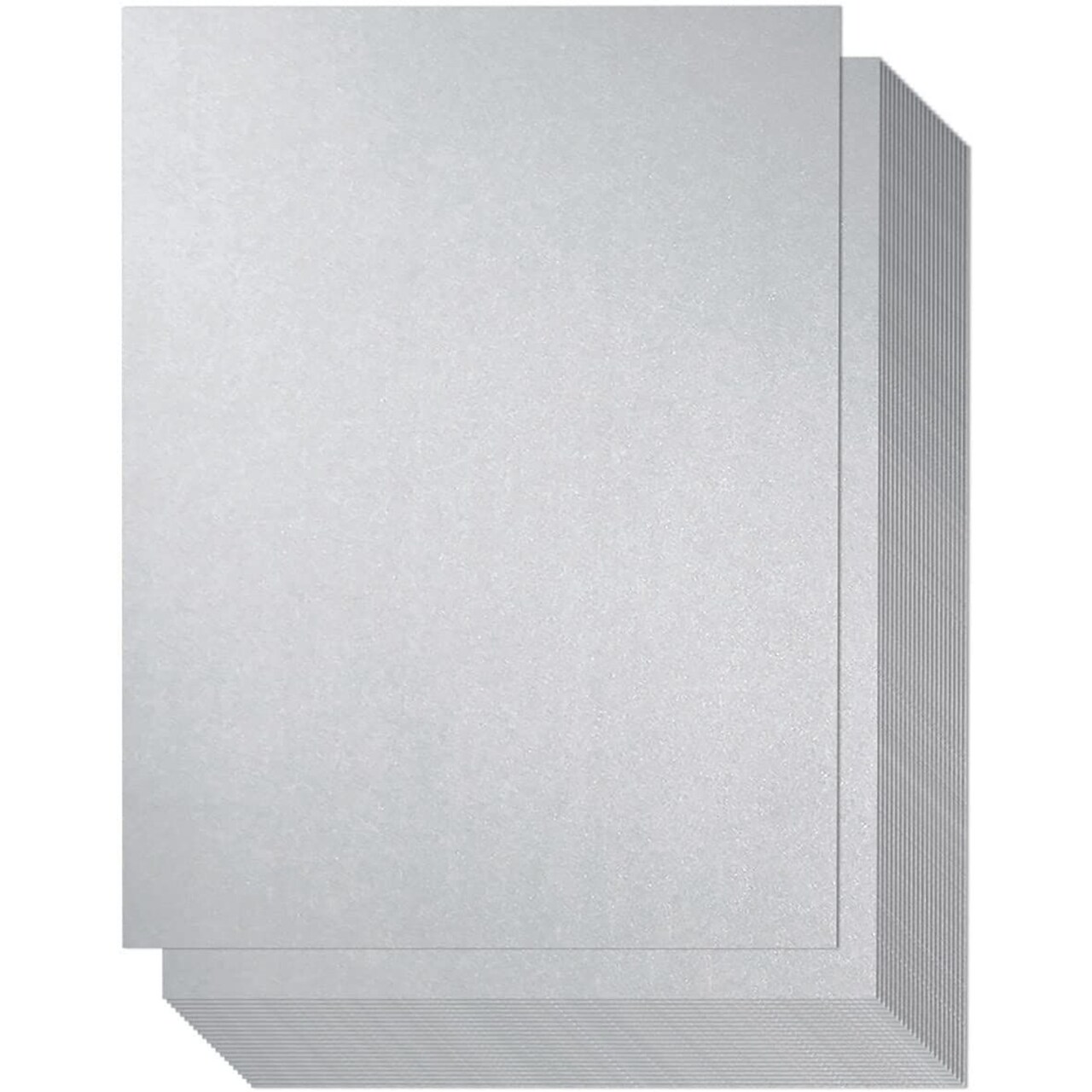This image is a computer-generated photograph intended for showcasing a product on a website for purchase. The product appears to be large gray building materials, possibly slabs of stone or gray quartz countertops, arranged in a neat stack. The background of the image is entirely white, highlighting the product. The stack consists of numerous rectangular pieces, all gray in color with subtle variations, possibly indicating different textures such as stone or cardstock. One piece on the top of the stack is slightly lifted and askew, drawing attention to the layered arrangement of the items. Shadows cast by the stack emphasize its depth and the number of items within it. The product is viewed from a downward angle, and despite the computer-generated nature of the image, it closely mimics a realistic presentation.